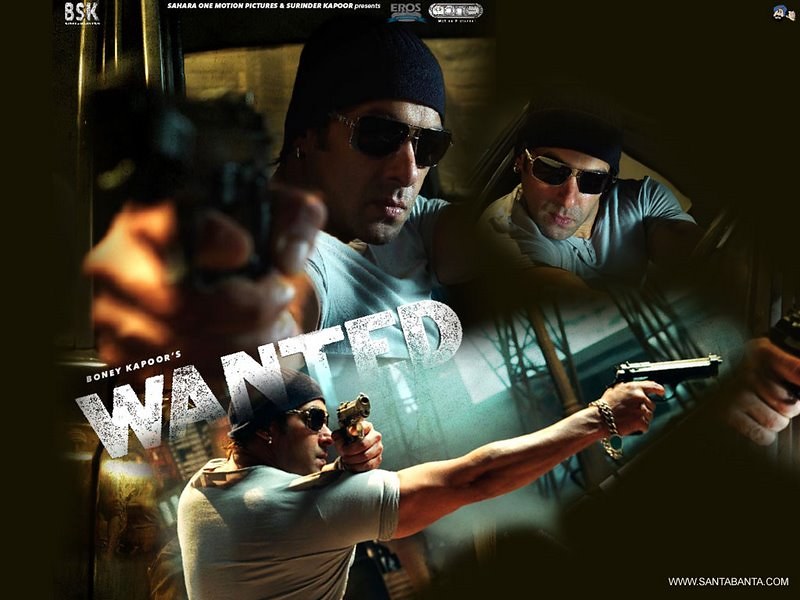The promotional movie poster prominently features a gritty atmosphere with an industrial background, consisting of a blurry gray brick wall and a dark, night sky. Positioned at the top left, the text reads "BSK Productions, Sahara One Motion Pictures, and Boney Kapoor Present." The central figure, appearing three times across the poster, is a man wearing a black ski cap, black square metal-framed sunglasses, and a white T-shirt. He is depicted in various intense poses: in one, he is inside a car, gripping the steering wheel with one hand and pointing a pistol with the other; in another, he is facing slightly left, aiming a gun toward the camera with his face in sharp focus while his hand and the gun are slightly out of focus; and in yet another, he holds two guns, one aimed outward and the other over his bicep.

The text "Boney Kapoor's Wanted" is prominently displayed diagonally across the center of the image in bold white capital letters. The man is also adorned with a silver bracelet featuring a green stone on his right wrist. The poster has distinct black borders around each image and displays the URL "www.santavana.com" in white text at the bottom right corner.